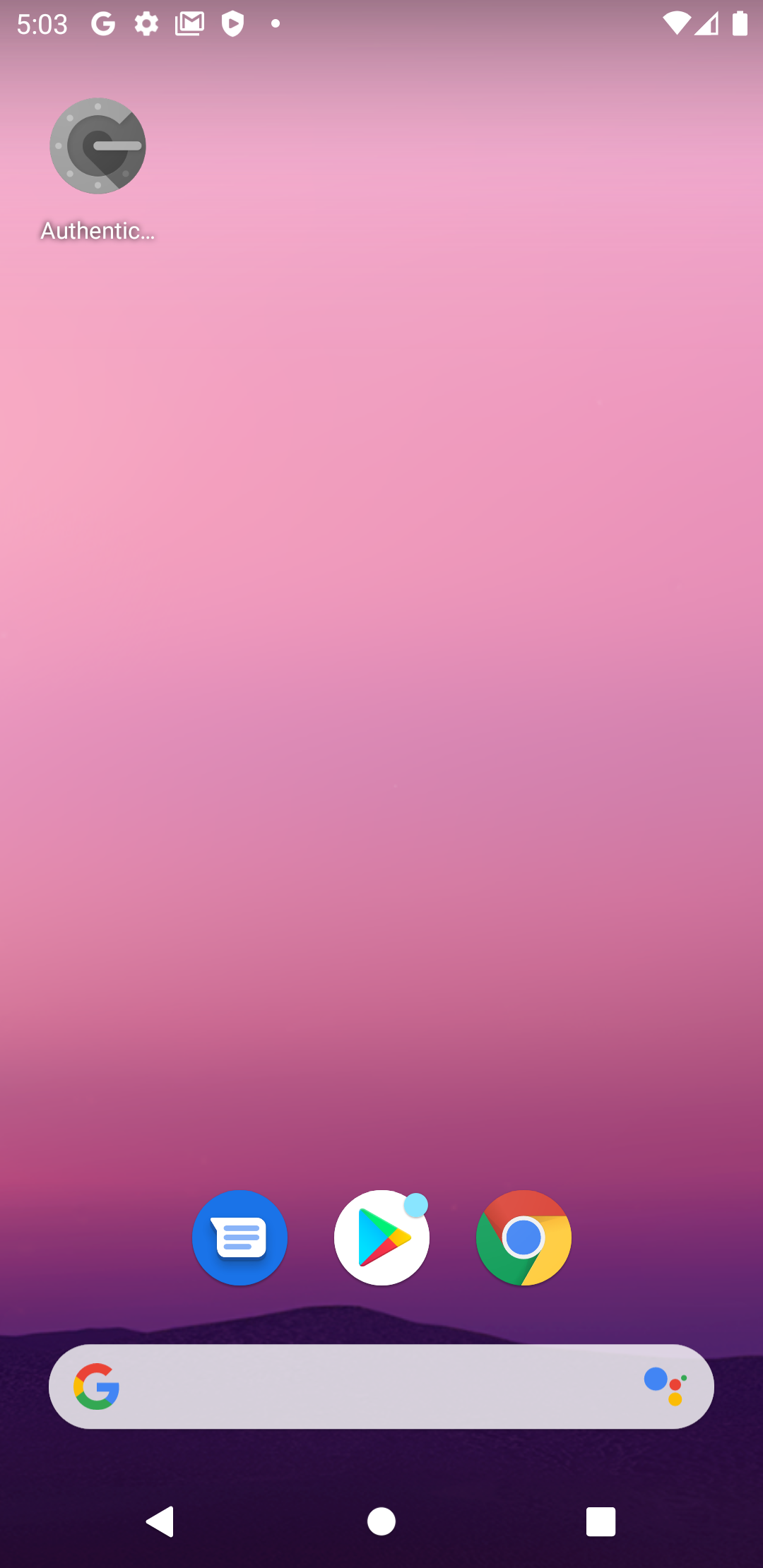Here is a detailed and cleaned-up caption for the image described:

"The screenshot captures the home screen of a mobile device. Dominating the top left corner is the Google Authenticator app, easily identifiable by its gray 'G' icon. The rest of the apps are situated towards the bottom of the screen, including the Messaging app, Google Play app, and Google Chrome. Directly beneath these apps lies the Google search bar, providing easy access to quick online searches. Below the search bar, the navigational buttons are prominently displayed: the back button, home button, and menu button from left to right. The background showcases a visually appealing pink gradient sky that seamlessly transitions into purple-hued mountains, adding a serene and picturesque touch to the home screen."